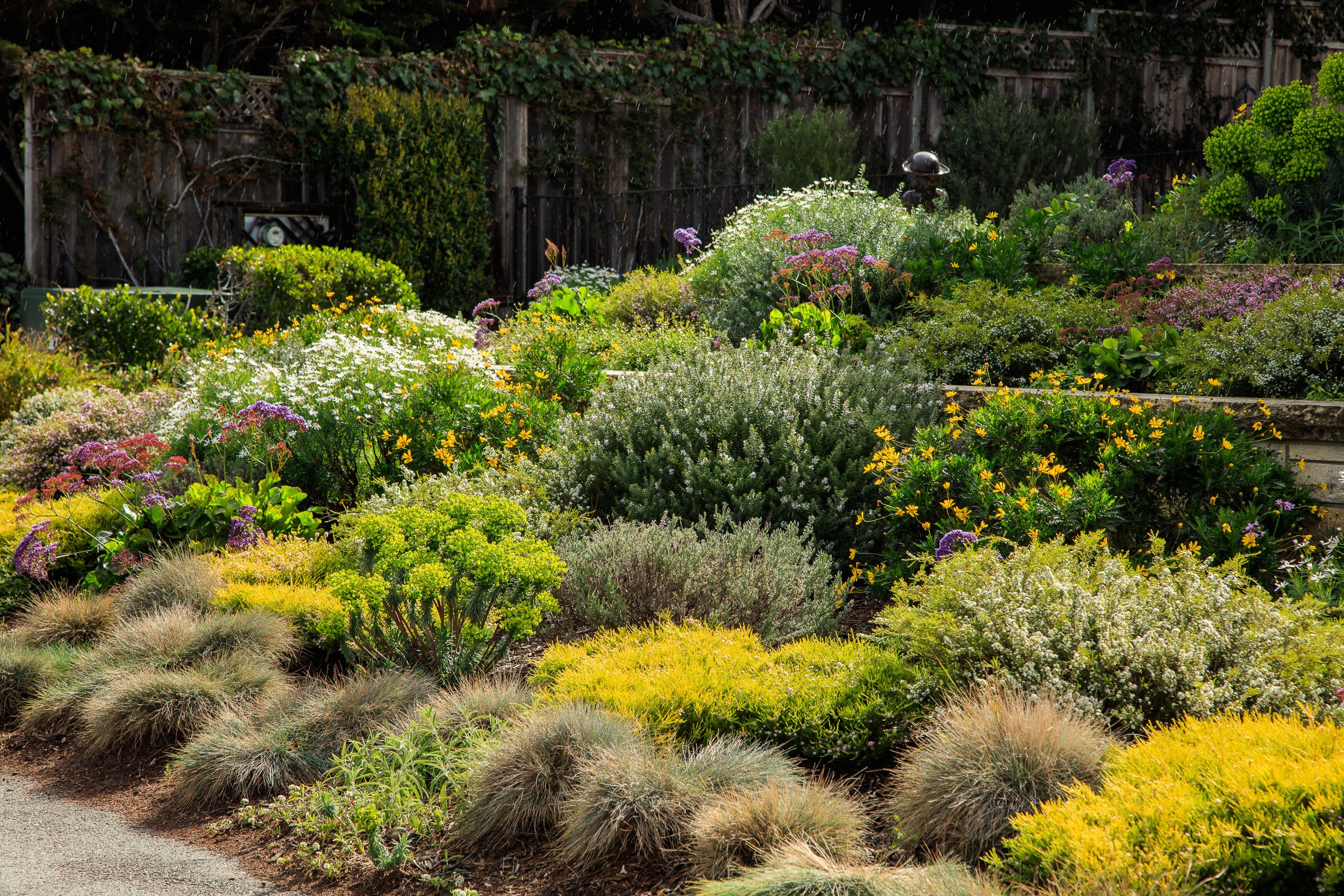This image is a detailed, daytime photograph taken outdoors in a garden. The garden is filled with a variety of vegetation arranged in a terraced structure. In the foreground, mostly unflowering plants that resemble tufts of fur, colored in gray and yellow, are visible. Moving towards the mid-ground, a colorful array of flowers extends from left to right, including pink, purple, greenish-yellow, white, and a small purple blossom.

Towards the back, the garden features three discernible rows of small flowers, with the top row predominantly white and yellow. Behind these rows, there's a wall or fence, with an upper terrace visible. This upper terrace contains more flowers—primarily purple—intermixed with soil, green bushes, and additional white flowers. 

In the top right-hand corner, a green bush can be seen. Further back, a tall, gray wooden fence is evident, adorned with creeping ivy and other climbing plants. Attached to this fence appears to be an electric meter. The garden is vibrant with colors, featuring yellow and green shades, various grasses, and brightly colored flowers.

Additionally, a person wearing a hat seems to be in the background, possibly near the upper terrace. The top right also features what looks like a statue of a man, partially hidden among the bushes. The entire scene exudes a private, well-maintained garden space, rich in diverse plant life.